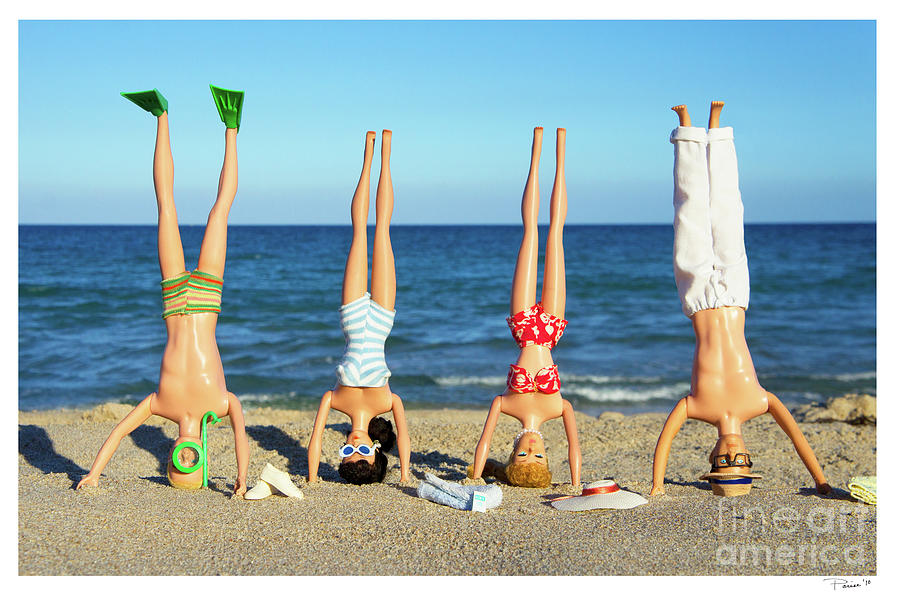The image is a horizontal, realistic photograph taken at a sunny beach, featuring a well-lit blue sky with scattered white clouds and a vivid blue ocean in the mid-ground. The groomed, yellow sand in the foreground is home to four Barbie-style dolls performing headstands, facing the camera, dressed in beach attire. From left to right: a blonde man in green swim trunks, green scuba goggles, and flippers, with a pair of white gym shoes nearby; a brunette woman in a blue and white striped bathing suit with matching sunglasses, next to a beach towel; a blonde woman in a red and white floral bikini, with her sun hat placed beside her; and finally, a man wearing white beach pants, a hat, black glasses, and equipped for a relaxed day. The image also features a watermark in the bottom right corner reading "Fine Art America" and is signed in black ink, though the signature is illegible.